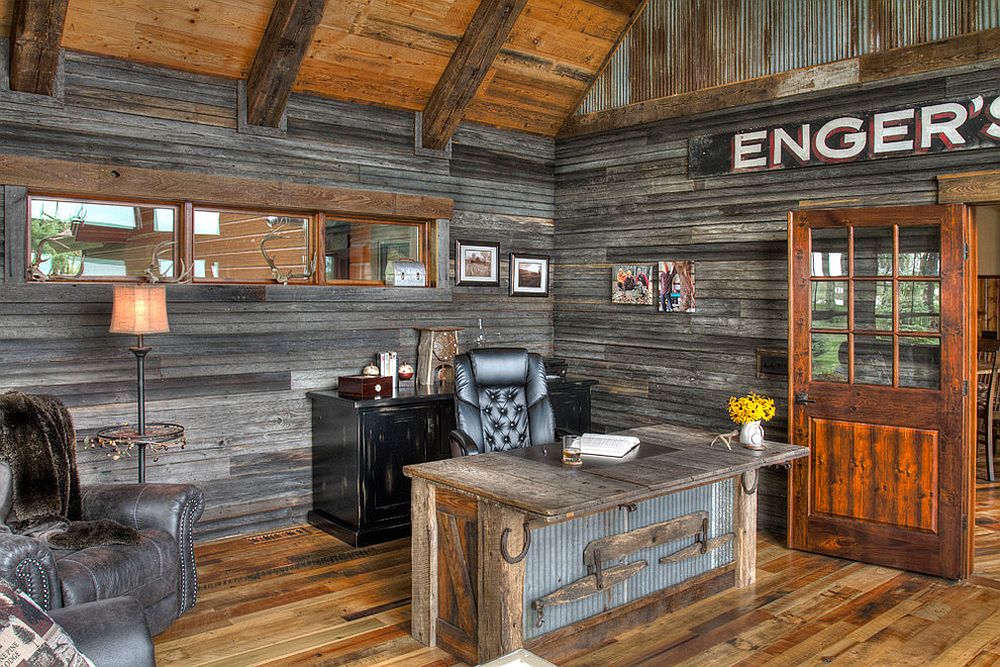The image captures the rustic charm of an indoor cabin-like setting, featuring weathered wooden walls and floors in varying shades of gray and brown. Overhead, the sloped ceiling boasts heavy wooden beams complemented by metallic accents. The ambiance of the room suggests a cozy office space, with an eye-catching black leather chair positioned behind a wooden desk adorned with metal accents. On the desk rests a white vase holding yellow flowers, an open book, and a glass of water. 

A black cabinet with indistinct details stands behind the chair. To the left, a recliner draped with a blanket adds comfort beside a lit brass lamp, which illuminates the nearby windows composed of three glass panes. The wall also displays an array of pictures, adding a personal touch to the space. Above a wooden door featuring nine clear window panes divided by wooden bars, a sign reads "Enger's" in white letters, reinforcing the rustic yet inviting atmosphere of this unique office.